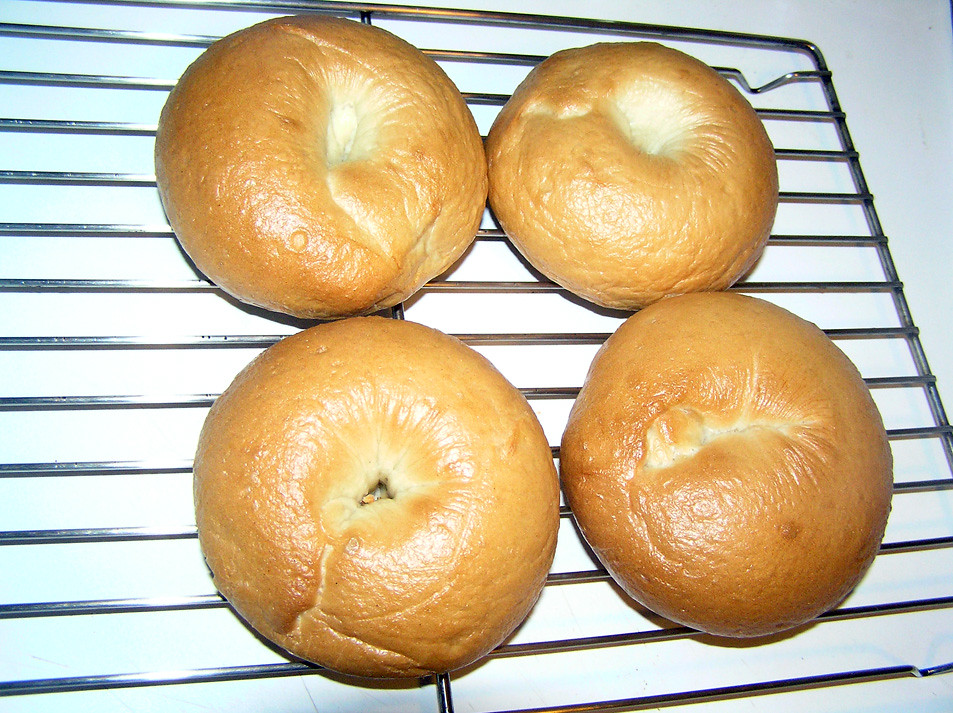The image showcases four freshly baked, golden brown bagels nestled on a silver, stainless steel cooling rack. The rack, positioned on a white countertop, has evenly spaced wires and a distinct indentation on one end to secure it in place. The bagels, with their characteristic small dimples in the center, sit in a neat arrangement—two atop and two below—with their fluffy, puffed-up appearance making them look especially enticing. Each bagel features a slightly unique navel-like depression on top, accentuating their homely, handmade vibe. Despite their resemblance to potential soup bowls, these round loaves are unmistakably dinner rolls, crafted from a white dough that has been perfectly toasted in the oven.